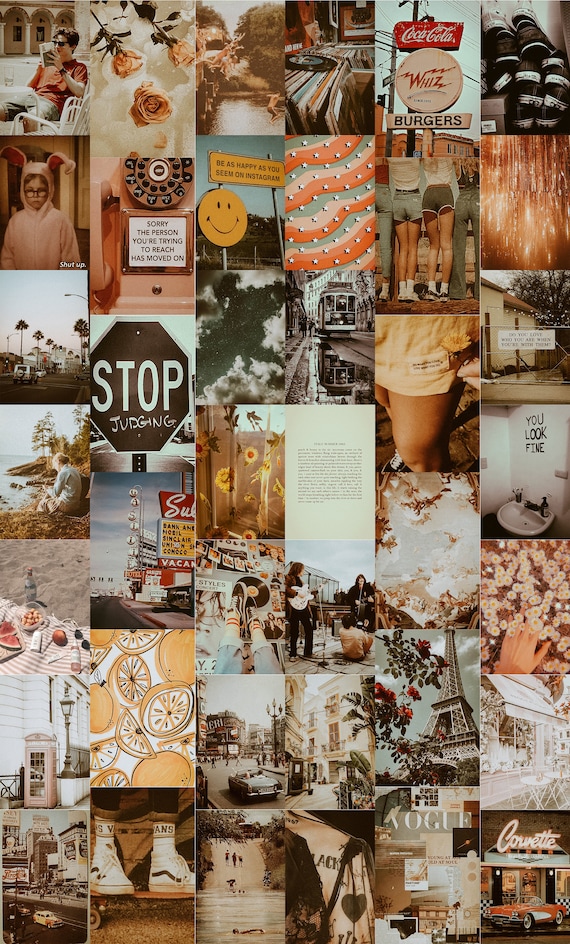The image is a vertical rectangle collage composed of approximately 40 individual portrait-oriented photographs arranged in a 6x7 grid. The color scheme predominantly features sky blue, orangey hues, and faded sepia tones with highlights of red, white, and gray. The photographs seem to capture scenes reminiscent of mid-20th century Americana, exhibiting elements like a vintage Corvette in front of a diner, and older Coca-Cola signs. Among the images, you'll find diverse subjects such as a man reading, roses on the ground, a smiley face sign, a stop sign with "stop judging" graffitied underneath, and a drawing of cut lemons. Additional photographs include a block of text, wildflowers, a pair of feet in sneakers, the Eiffel Tower, a little boy from A Christmas Story in a bunny suit, and people playing in a band on a stage. A few images depict road or business signs, a phone booth, and various city scenes. The overall theme evokes a nostalgic, vintage aesthetic with a collage of realistic and perhaps a few drawn images.